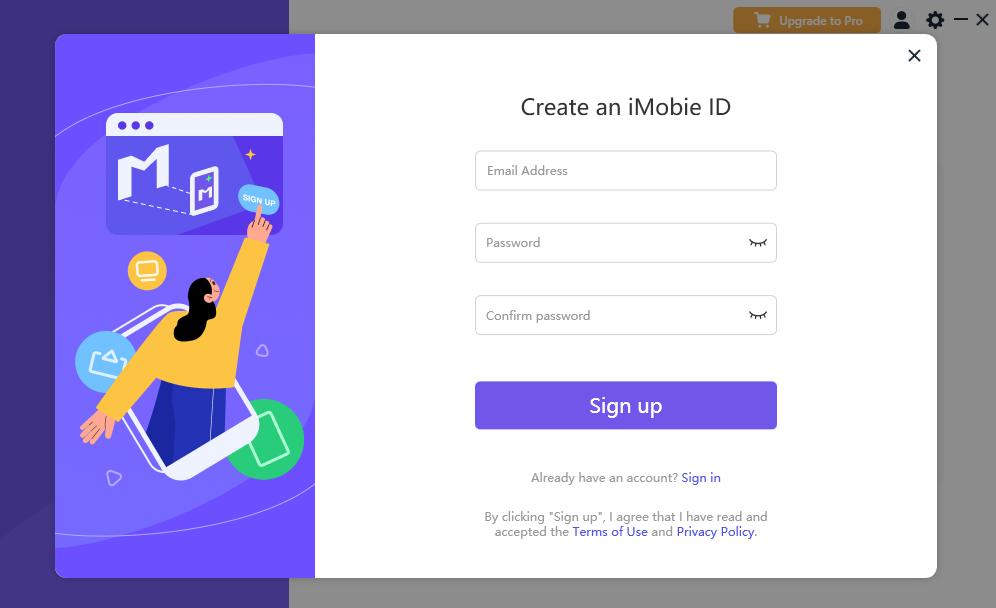This detailed screenshot displays the Create IMOB ID window, designed for user account creation. The interface comprises three text fields: one for entering an email address, another for the password, and a third to confirm the password. Below these fields sits a prominent purple "Sign Up" button. Beneath this button, the text reads "I already have an account," followed by an interactive "Sign In" link in purple. The lowest row of text states, "By clicking Sign Up, I agree that I have read and accepted the Terms of Use and Privacy Policy," with "Terms of Use" and "Privacy Policy" also highlighted in purple, contrasting with the rest of the gray text. This entire setup is placed against a clean white background.

To the left of this account creation form is a visually appealing graphic with a purple background. The graphic features an infographic-style illustration of a woman in an orange shirt and blue pants, emerging from a tablet screen. She is pointing at a browser window shown above her, which displays a blue "Sign Up" button at the lower right corner. The tablet screen also features various icons, including an orange computer monitor and another icon with a green background. The artistic style is non-photorealistic vector art, contributing to the modern and engaging design of the user interface.